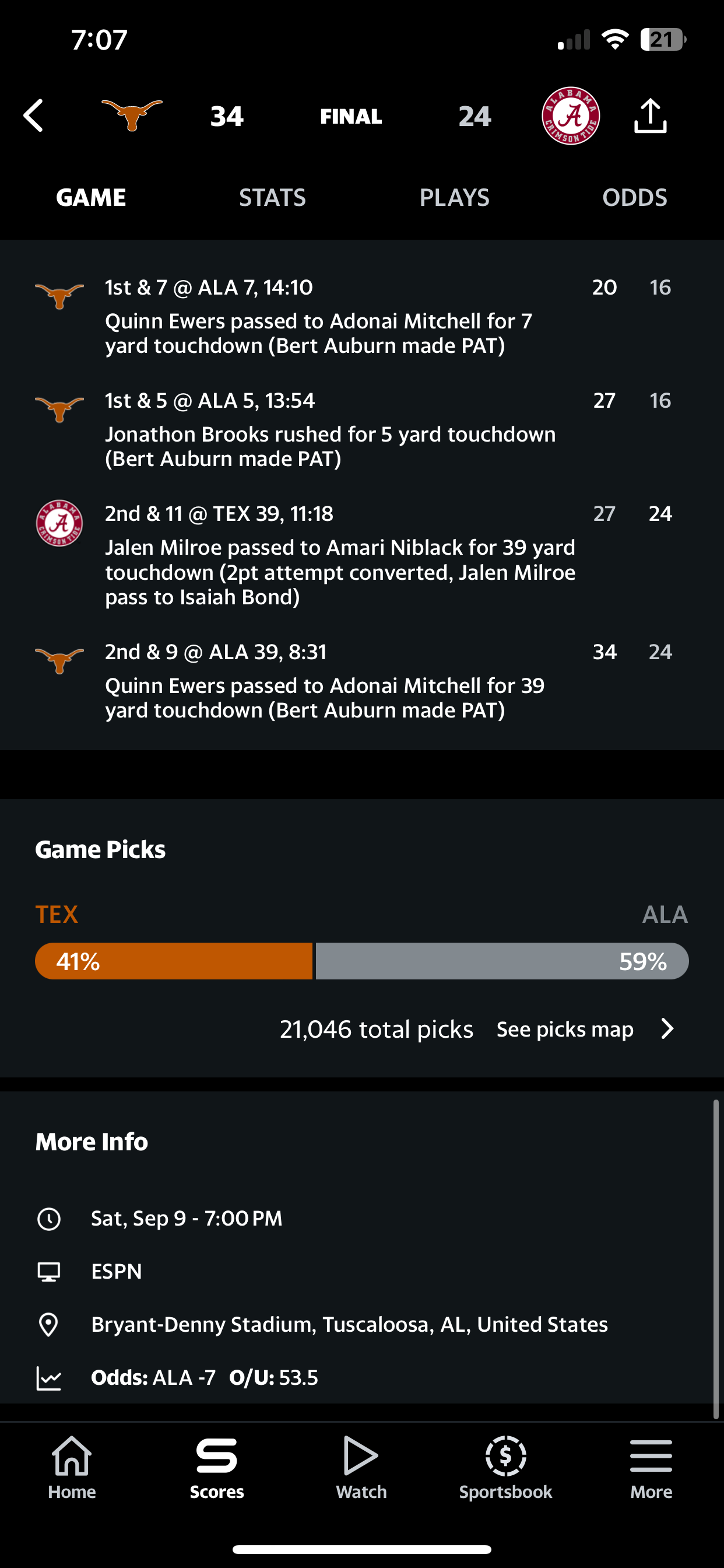Screen capture from a mobile device with a black background. At the top left corner, the time reads 7:07. Below the time, the screen displays various game statistics from a sports app. To the left, an icon of a bull's head in brown is shown next to a score of 34, indicating the final score. On the right, a red circular icon with a white center and a red letter 'A' is next to a score of 24. Underneath these icons, navigation options labeled "Game," "Stats," "Plays," and "Odds" are visible. The main section of the screen details game stats, starting with a notation at the top that reads "1st and 7 at ALA 7, 14:10," situating it just beside the brown bull head icon with horns.